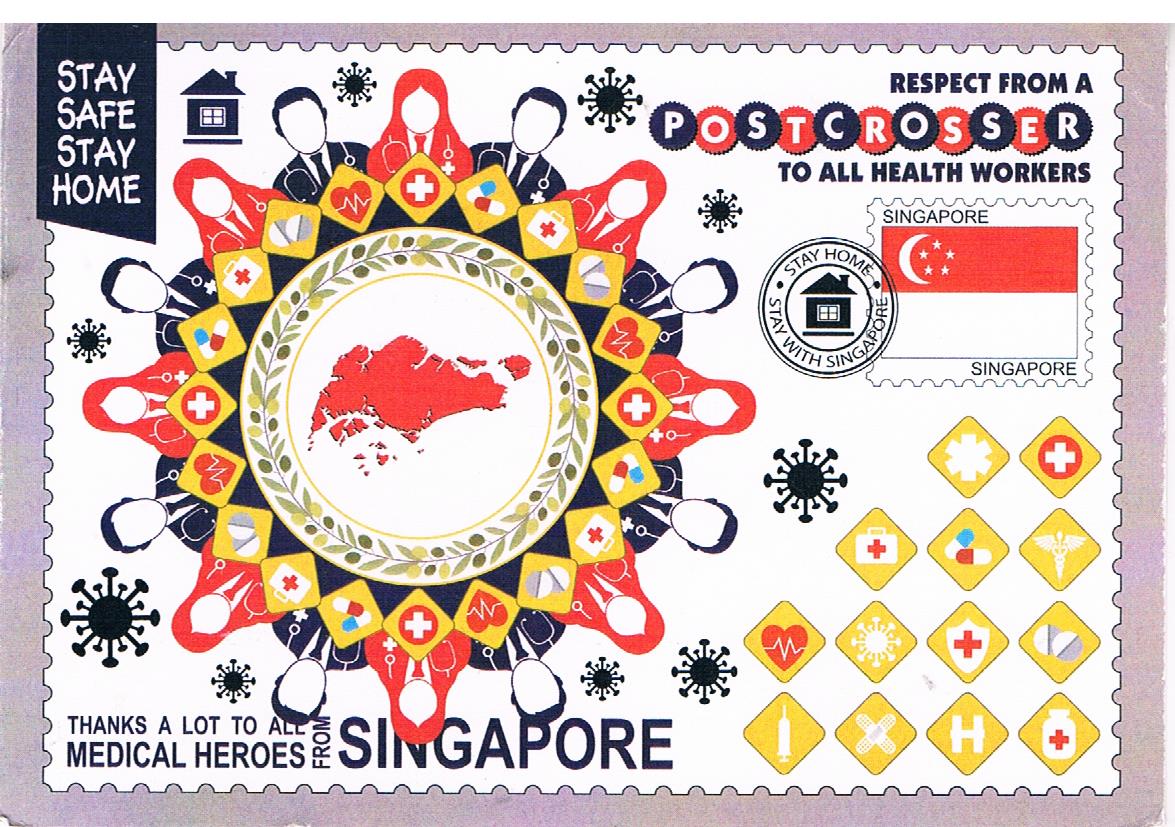The image is of a postcard with a light purple scalloped border and a white background, conveying a message of gratitude and solidarity. In the upper left corner, there is a blue banner with the text "Stay Safe, Stay Home" in white, accompanied by a hand-drawn graphic of a house. At the center of the postcard, a circular graphic features the red outline of Singapore, encircled by images of medical professionals clad in blue and red attire, interspersed with corona-style icons. Surrounding the circle is a laurel frame, symbolizing honor and victory. On the upper right side, the text reads, "Respect from a Post-Crosser to All Health Workers," with "POST CROSSER" presented in alternating black and red circles with white letters. Below this, there is a Singapore stamp showcasing the national flag and a postmark stating "Stay Home, Stay with Singapore." Alongside the stamp, from the center right to the lower right edge, is a pattern of yellow diamonds containing medical symbols. At the lower left edge, the text "Thanks a lot to all medical heroes" is written in black, with "medical heroes" in larger print. Vertically aligned text next to it reads "From Singapore."